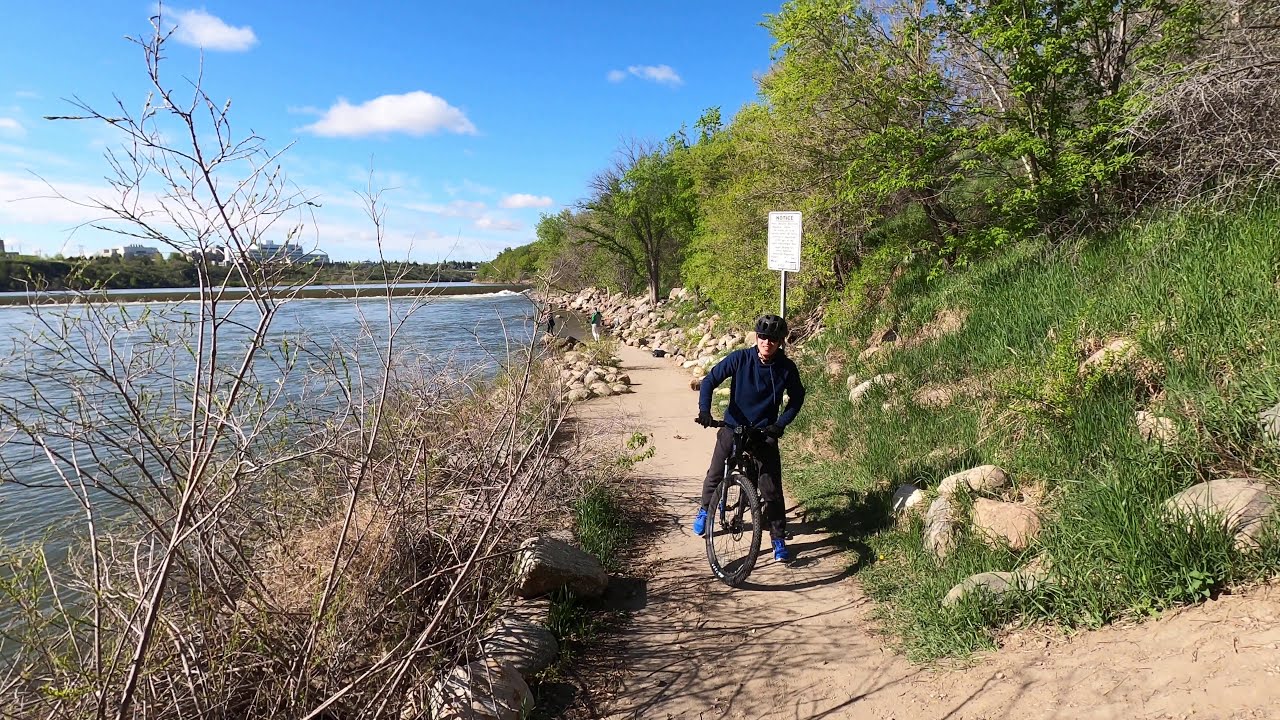A photograph taken during the daytime captures a man temporarily stopped on a black bike along a lengthy dirt path, which extends into the distance. The cyclist, outfitted in a black helmet, jacket, jeans, gloves, and bright blue sneakers, has his left leg resting on the ground and his right leg positioned on the pedal. The path is scattered with numerous rocks and boulders. To the left of the path, there's a waterway, likely a stream or a narrow man-made river, with blue water. The waterway features some visible waves or rapids, and possibly a bridge or dam further in the background. Across this waterway, trees line the opposite bank, along with some distant buildings visible in the background. To the right of the image, the terrain rises slightly to form a hill covered in green grass and deciduous trees, some of which have bare branches, suggesting an early spring setting. The scene is bathed in natural daylight, with a clear blue sky and white clouds visible in the upper left corner. The cyclist appears to be approaching a fork in the dirt path.